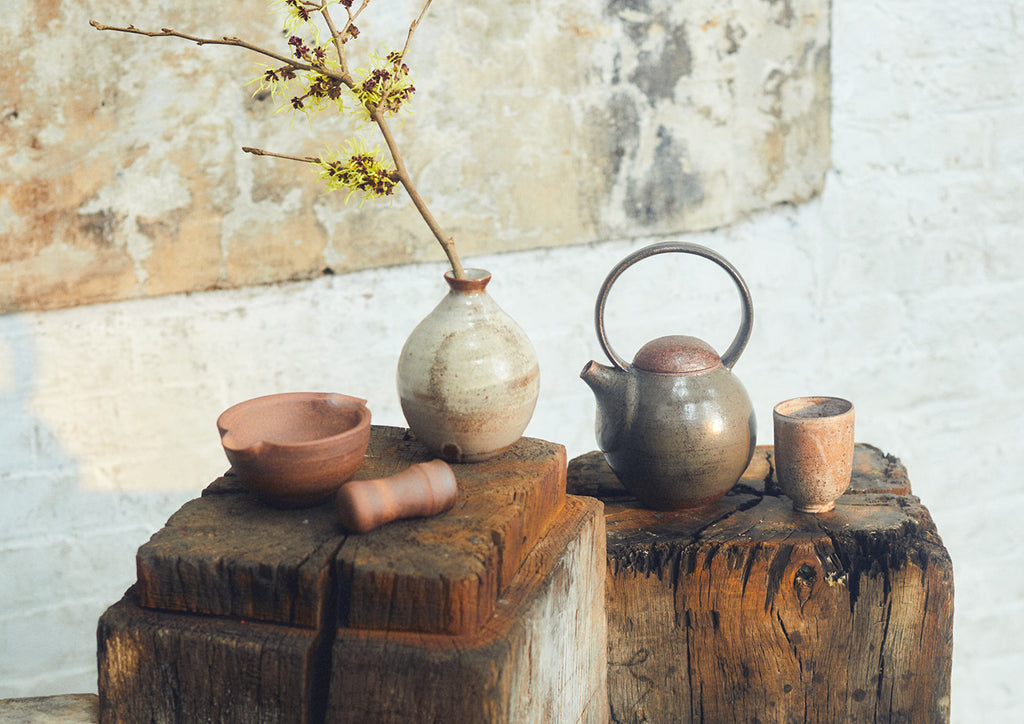The image captures a rustic and distressed arrangement of ceramic objects atop two weathered wooden blocks, set against a white brick wall with a tan and slightly darker tan abstract art piece in the background. The photorealistic scene includes a teapot with a large ringed handle and a cup, both made of fired clay, on the right wooden block. On the left block, there is a vase with dried flowers on a stick and a mortar and pestle, all crafted from the same pottery. The blocks are colored with various paints to enhance their aged appearance, complementing the overall aesthetic of decay and weathering.